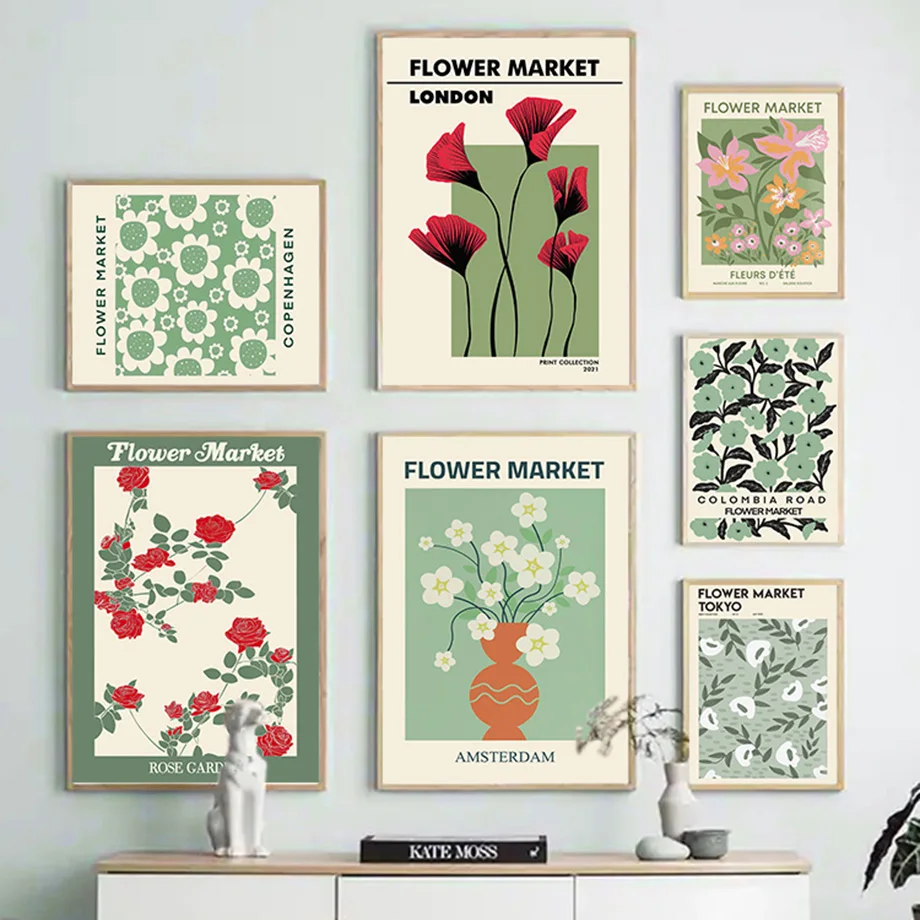The image showcases a meticulously arranged gallery wall in a minimalist home setting, featuring seven framed prints with light pine frames, each promoting a flower market from various cities. The top row houses two prints: the first one depicts the "Flower Market, Copenhagen" in green and white, adorned with daisies, while the second, beneath it, presents the "Flower Market, Rose Garden" featuring vibrant red roses against a green background. Intriguingly, a small lamb figure sits in front of these prints.

The next column begins with the "Flower Market, London," highlighted by red poppies on a green backdrop, followed by the "Flower Market, Amsterdam," which showcases petunias with a terracotta jug and a green background. Below these is a plaque reading "Kate Moss," nestled on a shelf. The final column includes the "Flower Market, Fleur de Tete," displaying lilies and primroses in shades of pink and orange with touches of yellow atop a green background, and the "Columbia Road, Flower Market," featuring dark green flowers.

Concluding the display, the "Flower Market, Tokyo," stands out with its soft sage green background and a vase containing white baby’s breath, accompanied by a stone and a small bowl. The wall art is complemented by a white credenza with a pine-colored top that supports a minimalistic décor, including a white vase with a plant, a white dog statue, a stone, a gray dish, and a black book titled "Kate Moss." The colors herein remain soft and elegant, dominated by greens, reds, oranges, and ivories, creating a harmonious and aesthetically pleasing display.